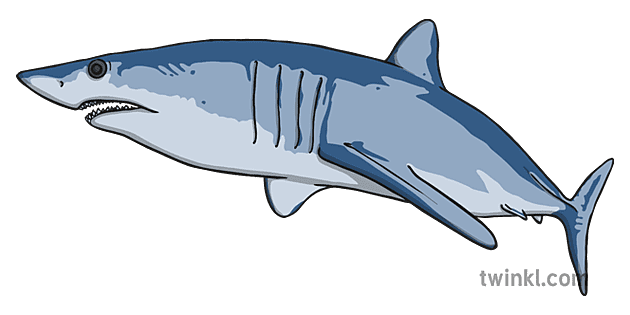The image is a simple, cartoon-style drawing of a shark facing the left side. The shark's top is dark blue, its middle section is light blue, and its underside is a light grayish-blue. It has a very pointy face with a slightly open mouth that reveals its sharp teeth. The shark features include a small dorsal fin on top, a small fin on the bottom, and a longer fin on the left side, with a black eye accentuating its face. The entire shark is the main focus, set against a completely white background with no other elements. Notably, the bottom right corner of the image displays the text "TWINKL.com," likely indicating the image's source. The overall impression is that of a simply drawn yet distinctly colored shark.